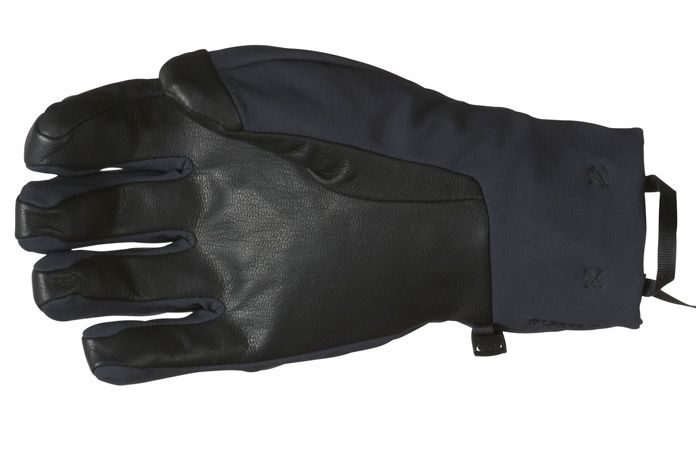This image depicts a single right-hand glove set against a white background, meticulously crafted from two distinct materials. The main body of the glove is a dark navy blue fabric, while the palm, the inner side of each finger, and the fingertips are reinforced with a black vinyl-like material. The glove features a loop at the right side of the wrist and another larger loop at its opening, designed to facilitate hanging or attaching the gloves together to prevent loss. The wrist area is detailed with two indentations; one on the upper side part and another on the lower side. Additionally, there is a small plastic tag near the wrist, possibly for branding or to clip the gloves together when stored. This glove's design suggests it might be used for either working or winter wear.